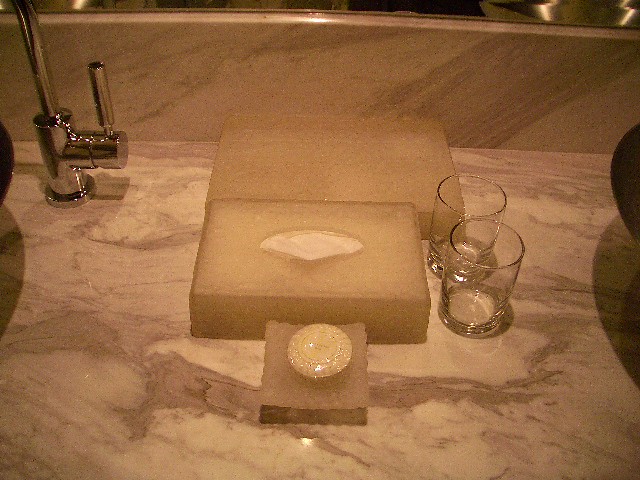The photograph features a sepia-toned bathroom countertop decked with an assortment of accessories. Two raised bowl sinks, positioned side-by-side, dominate the scene, flanked by shadows suggesting the presence of a soft light source. On the upper left, a sleek faucet and its handle, responsible for dispensing hot or cold water, accentuate the modern aesthetic.

To the right of the faucet sits a flat, ivory-colored container, potentially holding small items like q-tips, and adjacent to it, a rectangular tissue box. An exfoliating sponge, topped with a round bar of soap wrapped in cellophane, adds a touch of practical elegance. Two small drinking glasses further adorn the countertop, which is crafted from a beautifully patterned brown and ivory marble.

Just below the mirror, a subtle marble molding adds a sophisticated touch to the scene, with the mirror itself faintly visible along the photograph's upper edge, hinting at the room's reflective elegance.